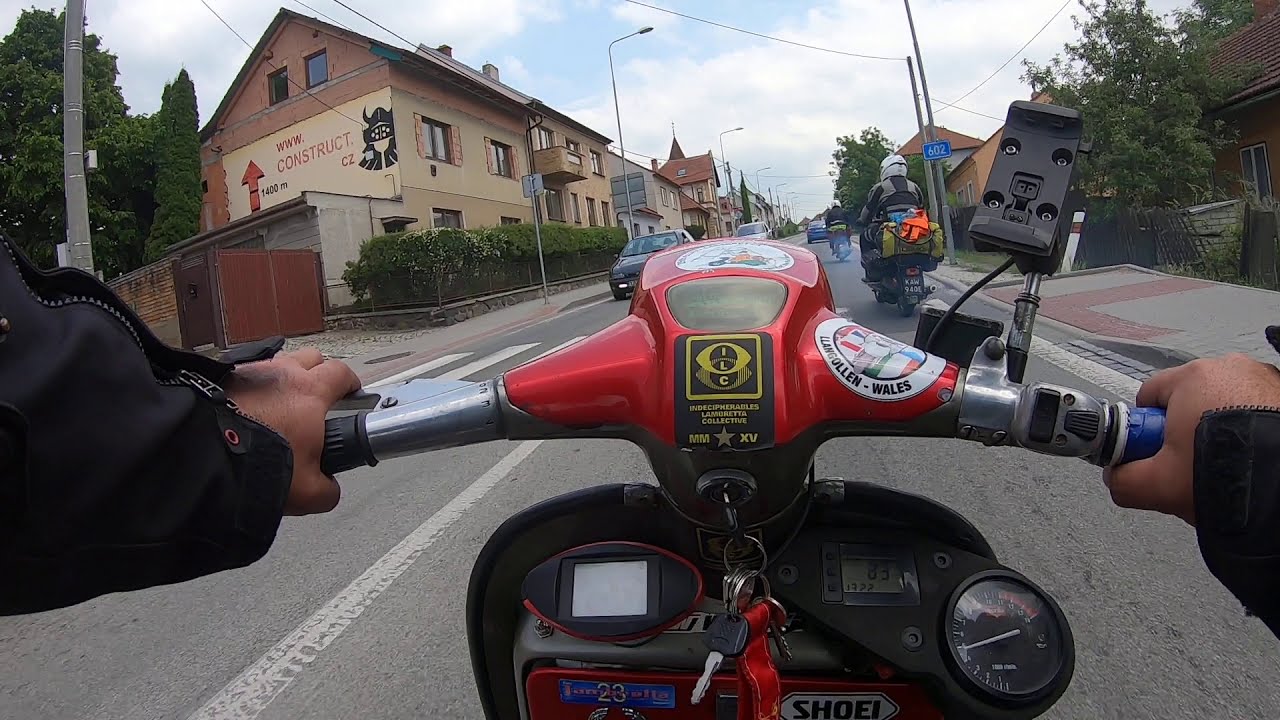This image is a first-person perspective from someone riding a red motor scooter down a quiet street. The scooter features black accents on the gauge holders, a black left handlebar, and a blue-marked right handlebar. There are various tags and stickers on the scooter: one in Welsh and another with "ILC" within an eyeball shape. The rider is wearing a black jacket and there's a phone holder on the upper right part of the handlebars. 

The street stretches out for several blocks with a few cars approaching from the left. The rider is following two other mopeds, one of which has a yellow pack, and a car leading them. To the left, rows of tan, beige, and brown buildings line the street, the first adorned with a sign that reads "WWW Construct CZ," pointing forward with an arrow and featuring a Viking helmet stencil image. A row of dark green hedges stands in front of this building. Additionally, there's a blue street sign with the number 602 visible to the middle right. Trees can also be seen on the right side of the image, contributing to the serene atmosphere of the scene. The overall impression is of a leisurely ride through a calm, possibly Welsh, urban area.